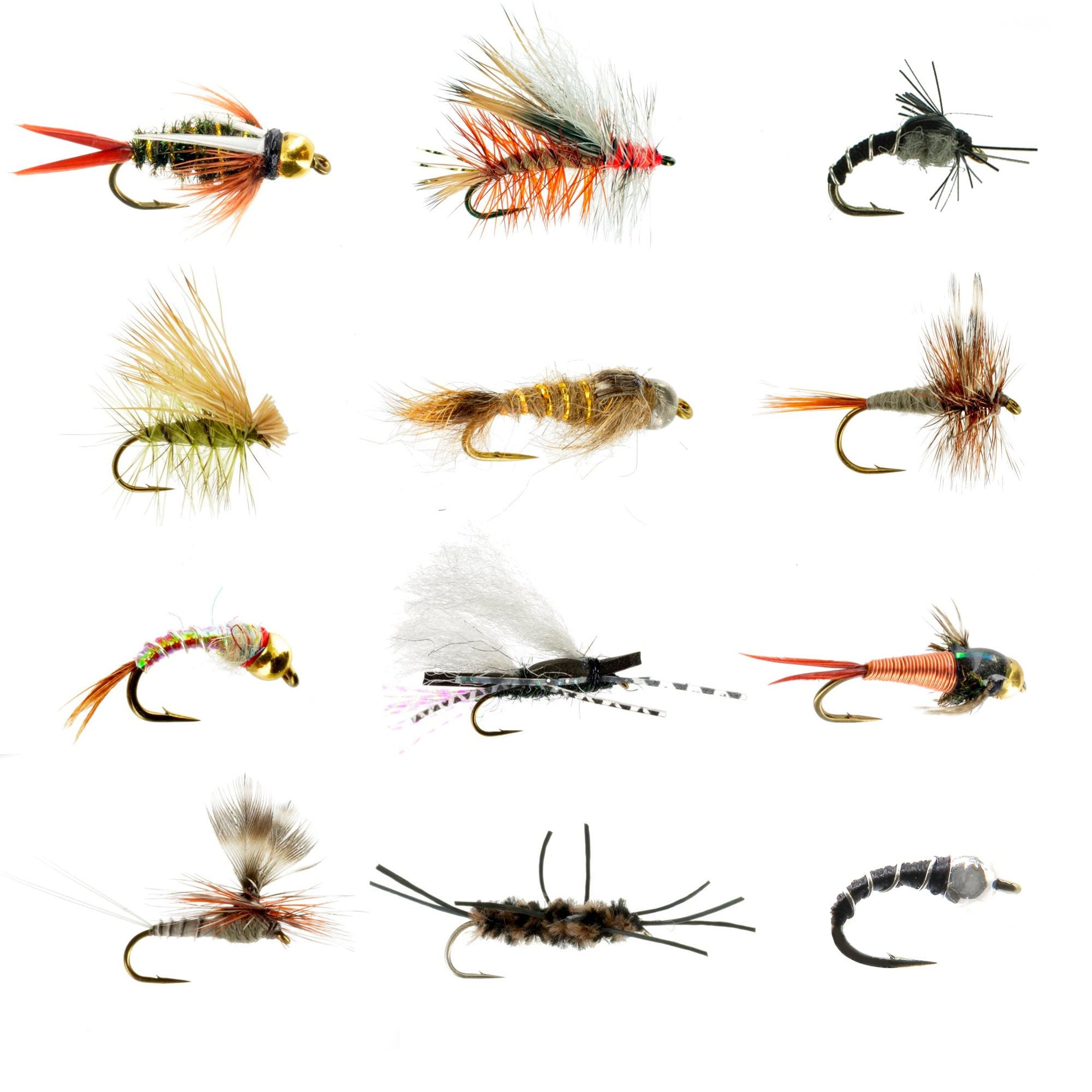The image showcases an array of 12 elaborate fly fishing hooks, organized in a grid with three columns and four rows. Each hook features distinctive designs, mimicking the appearance of various insects to attract fish. While all hooks have a common structure, with a hook at the end ready to catch unsuspecting fish, they exhibit a wide range of styles and colors, such as black, orange, tan, and multicolored. The hooks have fur, hair, or feathers extending from them, enhancing their insect-like appearance. Some hooks have spiky or pointed ends, while others have wings that vary in length. The flies differ in their body structure as well; some have long or short tails, some are thick and furry, while others are thin or tightly wrapped in twine, without any apparent body. Notably, one fly features a feathery Mohawk-like design, adding a humorous touch to the collection. Despite their variance, each fly meticulously replicates the look of a bug, making them enticing bait for fly fishing.